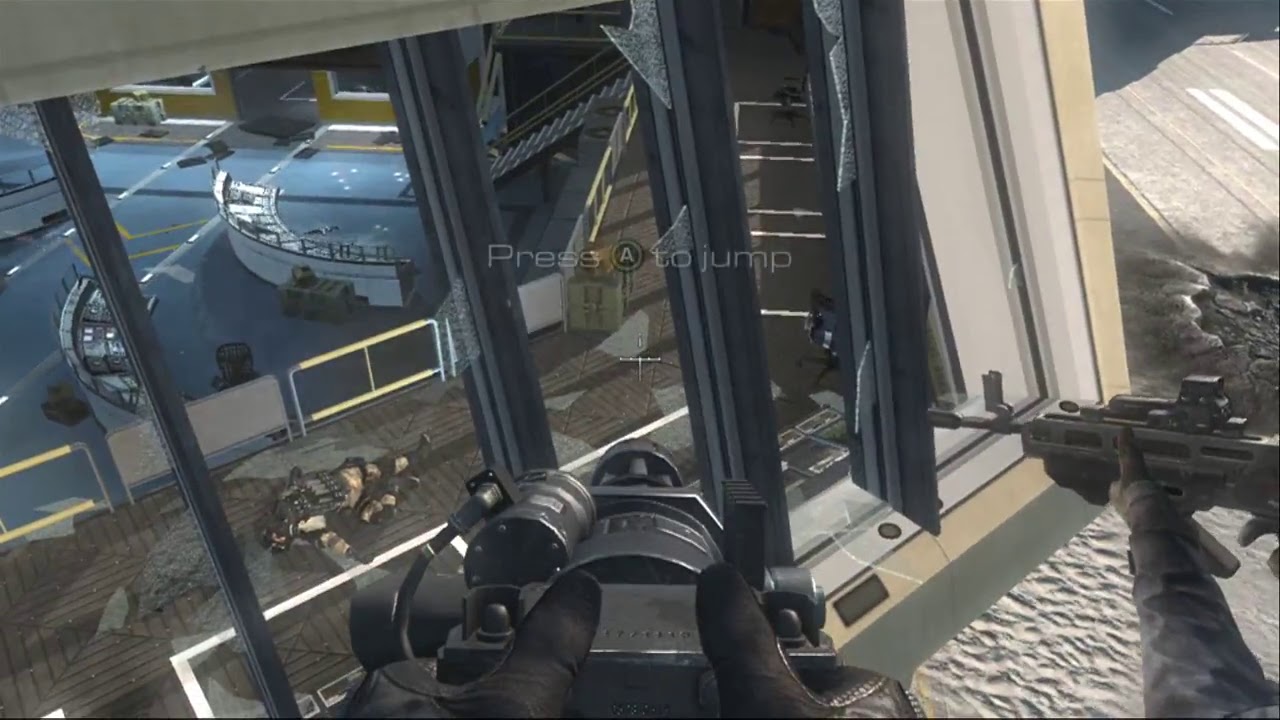The image is a highly detailed screenshot from a first-person shooter video game, presented from the player's perspective. In the foreground, the player's black-gloved hands grip a formidable black machine gun, aimed outwards. To the left, another character's camouflaged arm, also equipped with a semi-automatic or automatic rifle, is visible. The scene is set in an indoor environment with the players looking through shattered windows bordered by dark frames atop what appears to be sandy ground with visible ripples. The structure they are observing from an elevated vantage includes a brown upper walkway and a lower blue area filled with desks, consoles, and various floor markings, interconnected by stairs. A sprawled body clad in brown clothing and black military gear is noticeable on the upper deck. The ambiance of the scene is dominated by beige, gray, and faint yellow tones, illuminated by natural light, suggesting it is daytime. Centrally positioned on the screen is a faint, white text prompt "Press A to jump," indicating the next action required in the game.